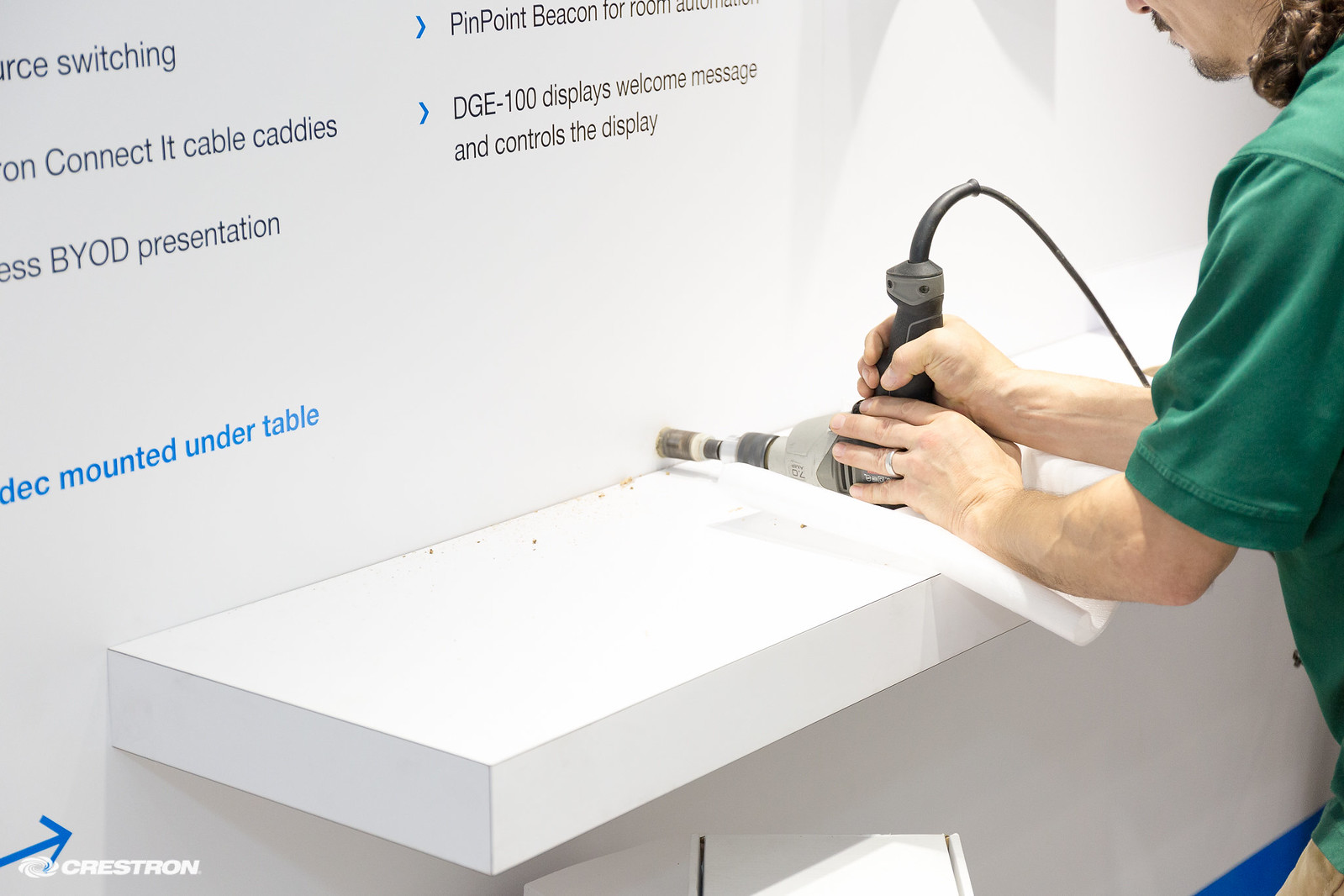In this indoor, rectangular photograph taken in the middle of the day, a man of Caucasian descent wearing a green short-sleeved shirt and a wedding band on his left ring finger is positioned on the right side of the image. He has a mustache, some chin whiskers, and longer hair draping over his shoulder, though the top of his head is cropped out of the picture. The man's arms are bent at the elbows as he uses a corded drill, held upside down with the handle facing upward. The drill, equipped with a circular hole-cutting attachment, is being used to make a hole just above a white floating shelf that extends from a white wall. A power cable extends from the drill handle, bending toward the right.

On the white wall, numerous text elements and blue arrow bullet points are visible, although they are not very legible or significant for reading out loud. In the upper left-hand corner, black text reads "source switching." To its right, a blue arrow points to "Pinpoint Beacon for Room." Below that, additional text, interrupted by arrows, continues with "on connect it cables caddies" and "DGE-100 displays a welcome message and controls the displays." The photograph features a color palette including black, white, blue, gray, green, and tan. The scene is framed to emphasize the man's work and the floating shelf at the center of the image. Additionally, in the bottom left corner of the wall, a watermark reading "Crestron" and a blue arrow pointing upwards are present.